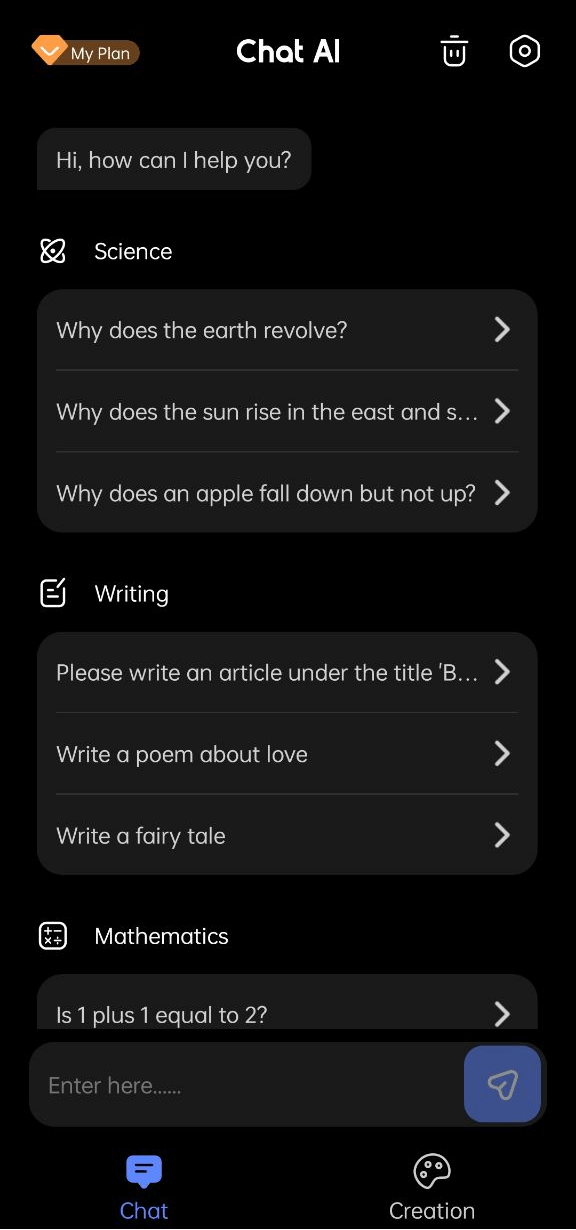The image appears to be a screenshot of a mobile application interface on someone's phone. In the upper left corner, the label "My Plan" is visible. At the top center of the screen, "Chat AI" is displayed, and to the right, there are icons for a trash can and a gear, indicating options for deletion and settings respectively. The background is entirely black.

In the middle of the screen, there is a text bubble that reads, "Hi, how can I help you?" Below this, an icon of a rocket ship with a ring around it signifies a section labeled "Science." Under this heading, there are three selectable options: "Why does the Earth revolve?", "Why does the sun rise in the east?", and "Why does an apple fall down but not up?"

Following the science section is a writing section, marked by an icon representing a document with lines and a pencil. This section offers three prompts: "Please write an article under the title 'B...'", "Write a poem about love," and "Write a fairy tale."

Next, there is a mathematics section, indicated by an icon of a square containing an "X" and a plus sign. This section includes a single question: "Is one plus one equal to two?"

At the bottom of the screen, there is a text input box labeled "Enter here," and at the very bottom, there are two buttons labeled "Chat" and "Creation."